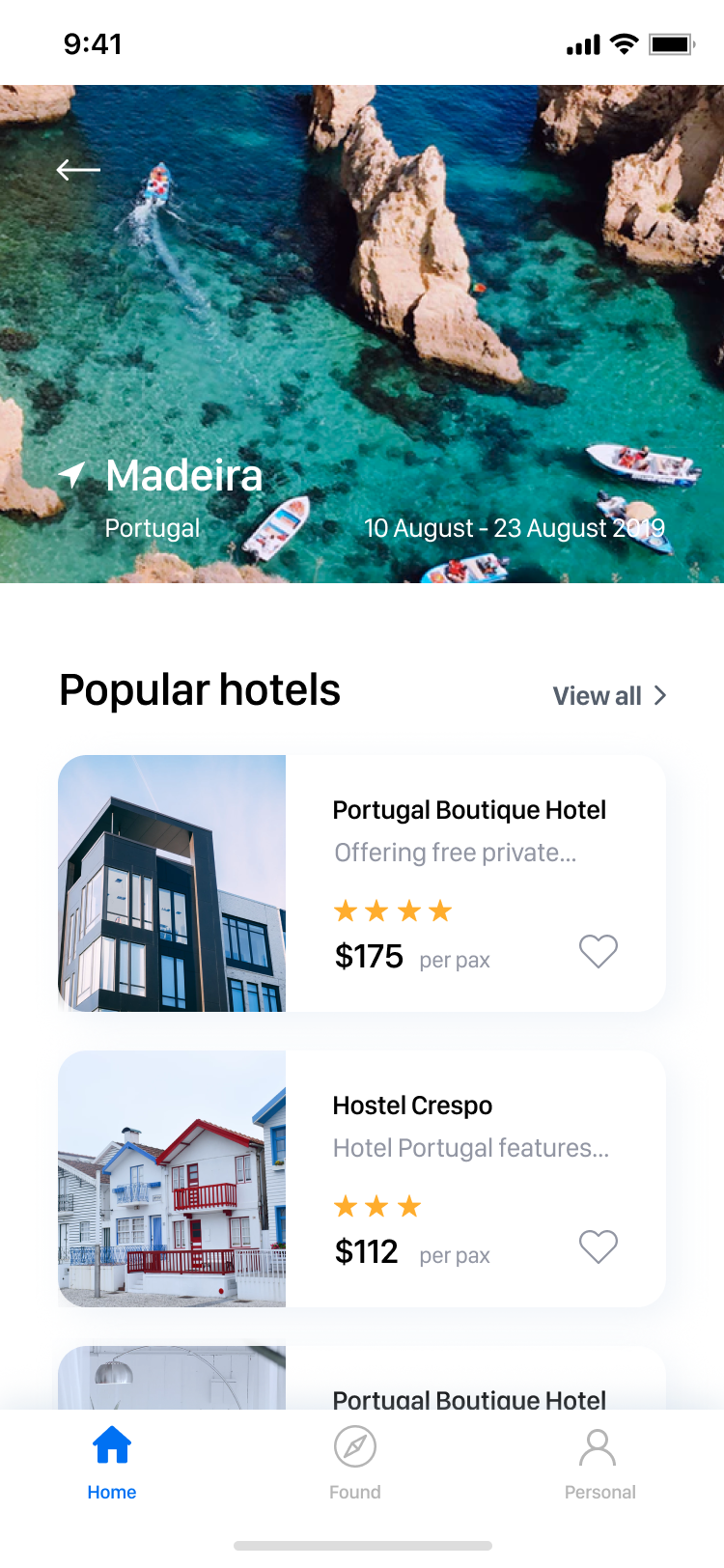This screenshot depicts the Home page of a travel or hotel booking app displayed on a smartphone. The top of the screen shows standard smartphone icons, including the time, battery level, and signal strength. Dominating the upper section of the app is a stunning image of a shallow ocean area, complete with several boats and towering rocks, creating an inviting marine scene. The text "Madeira, Portugal, 10th August to 23rd August, 2019" indicates the travel destination and dates.

Further down, there is a section titled "Popular Hotels" with an option to "View All" or scroll through the listings. Two hotel options are visible: "Portugal Boutique Hotel," priced at $175 per night and rated four stars, and "Hotel Crespo," priced at $112 per night with a three-star rating. Both listings include a heart icon, suggesting users can favorite them for future reference. 

At the bottom of the screen, there are three main menu icons labeled "Home," "Found," and "Personal," with the "Home" icon currently highlighted, indicating the active page. This detailed layout provides a comprehensive view of the app’s user interface focused on hotel selection.